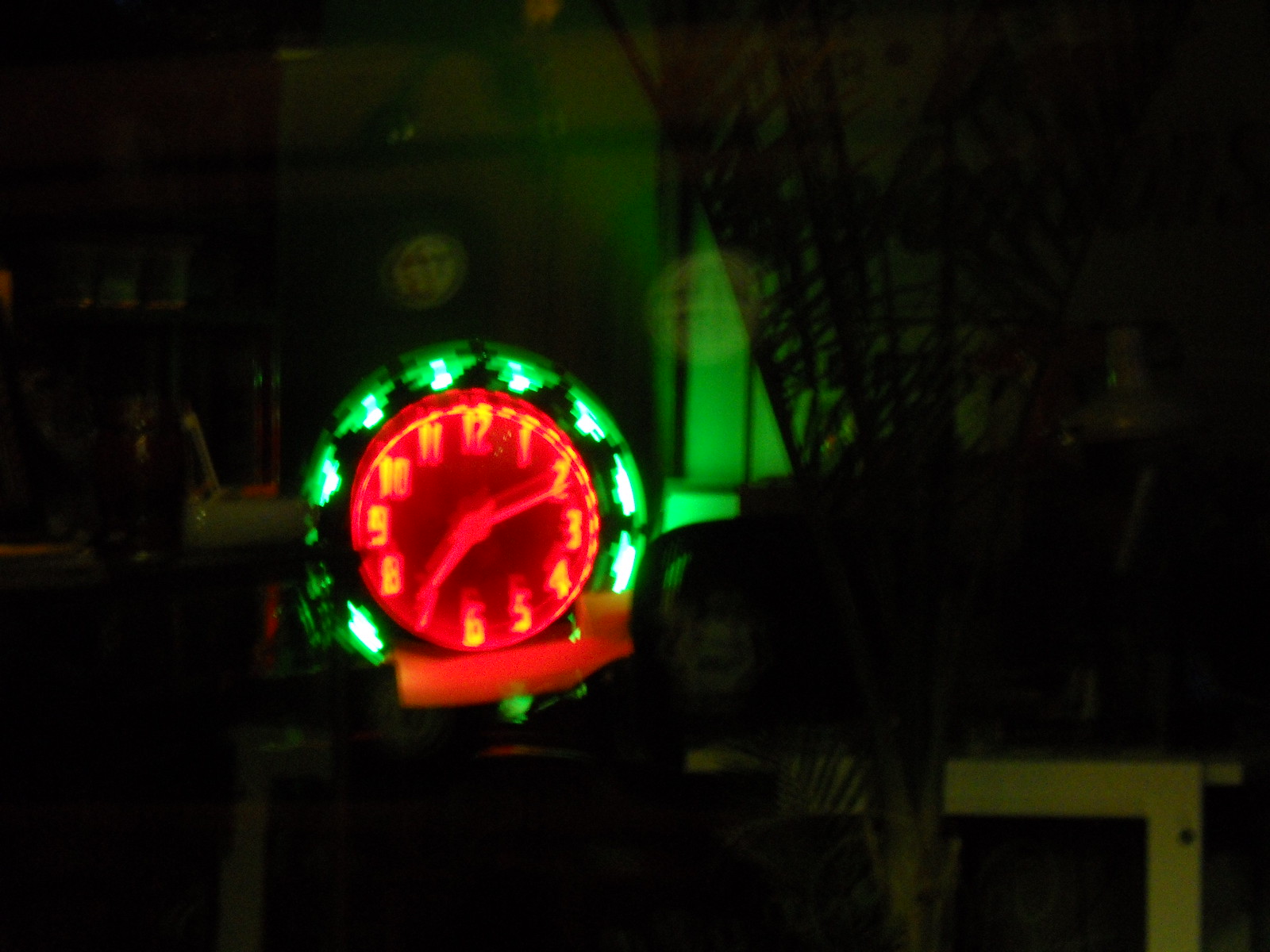The image depicts a vibrant circular cloth adorned in green and red hues, with a blurred, double-exposure effect suggestive of a camera shake. The outer ring features intermittent green sections interspersed with gaps, creating a segmented appearance. The center of the cloth is predominantly red, with illuminated numbers ranging from 4 to 12 encircling it. In the lower right corner, a peculiar face reflects in a mirror, characterized by a white complexion and black strands draping across it. Additionally, a black, semi-transparent cloth hangs from the ceiling to the right. On the left side of the composition, a white cloth is visible, featuring cut-out numbers.